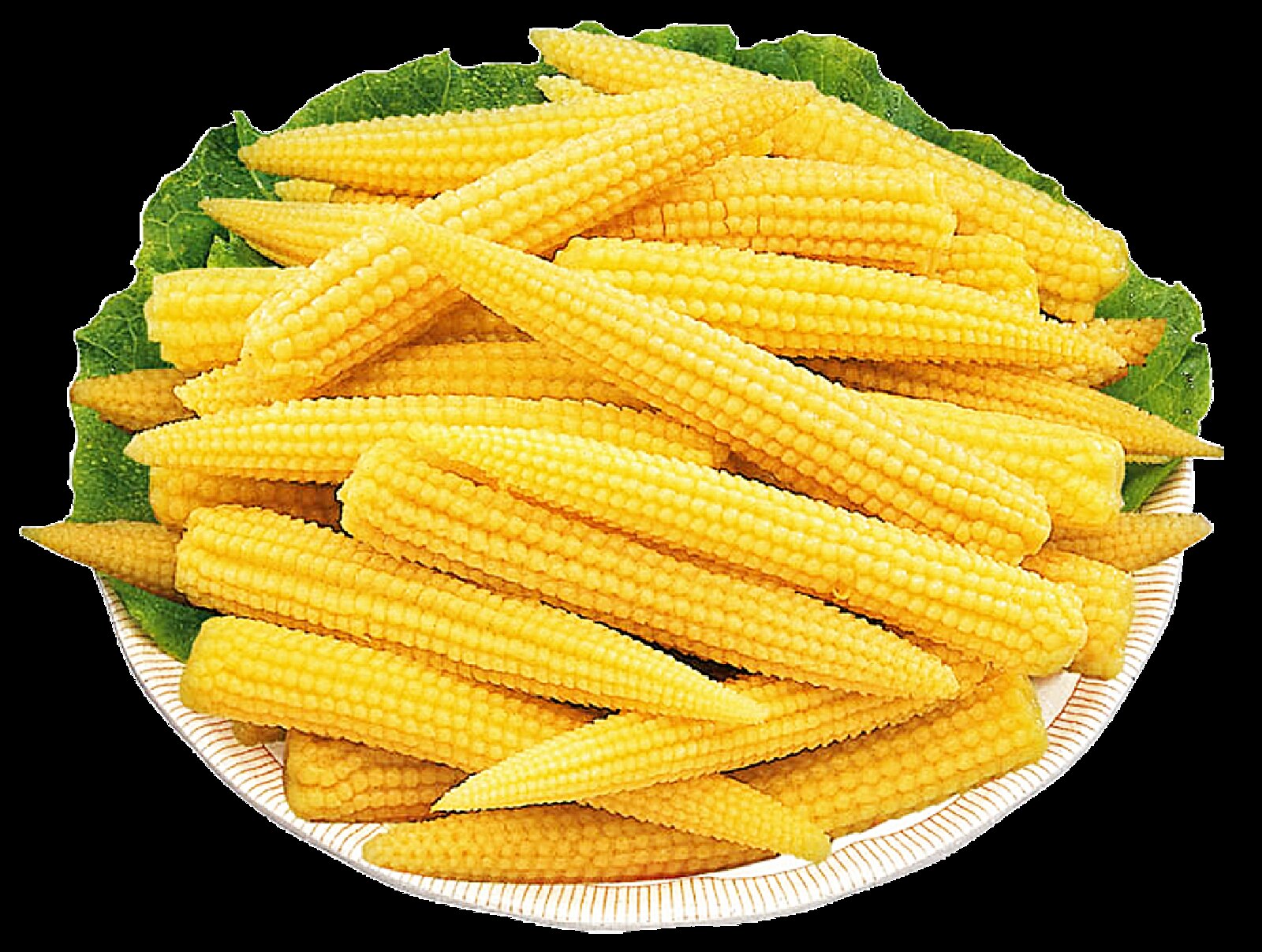This is a large, close-up square image with a solid black background that is mostly visible in the corners and slightly along the edges. The centerpiece of the picture is a white paper plate featuring a tight reddish-orange striping along the border. Piled high on the plate are approximately 25 narrow, long ears of baby corn, arranged in a somewhat haphazard manner with some pointing left, others right, and various angles. The bottom half of the plate is more visible, showing its ribbed edge, while the top half is mostly covered by a bed of green romaine lettuce leaves that create a natural, leafy border. One of the baby corns in the foreground has a distinctive white tip, but the majority are yellow. This composition is striking due to the vivid contrast between the bright plate and corn against the deep black background.